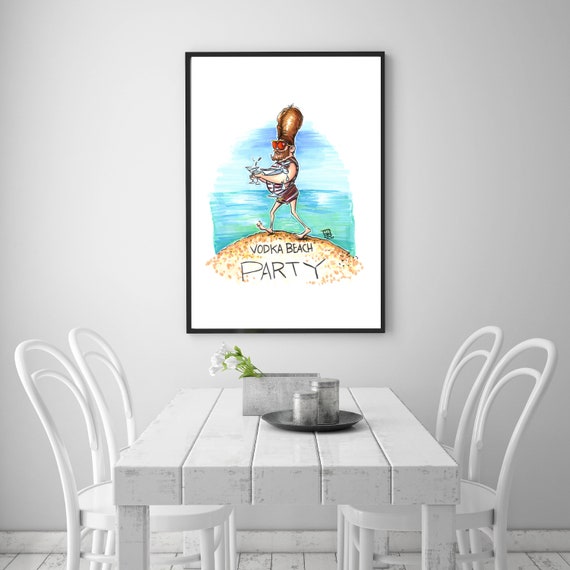The image depicts a minimalist dining room with a light grayish-white wall and matching white flooring. Central to the room is a sturdy, painted white wooden table flanked by four white chairs, with metallic backrests and possibly plastic seating surfaces. The focal point of the table is an aluminum box holding a single white flower, accompanied by a plate carrying two aluminum jars. Above the table, a prominently large, black-framed art piece captures attention. This illustration portrays a beach scene with blue sea and sky, featuring a comically large-headed man sporting a tall hairstyle, a long brown beard, and red sunglasses. The man, adorned in an old-style swim suit and a blue tie with a crocodile on his shoulder, holds a dripping cocktail glass while standing on yellow sand. Etched at the bottom of the scene, in capitalized handwriting, are the words "Vodka Beach Party." The combination of white elements throughout the room alongside the vibrant, detailed poster creates a stark and engaging contrast.